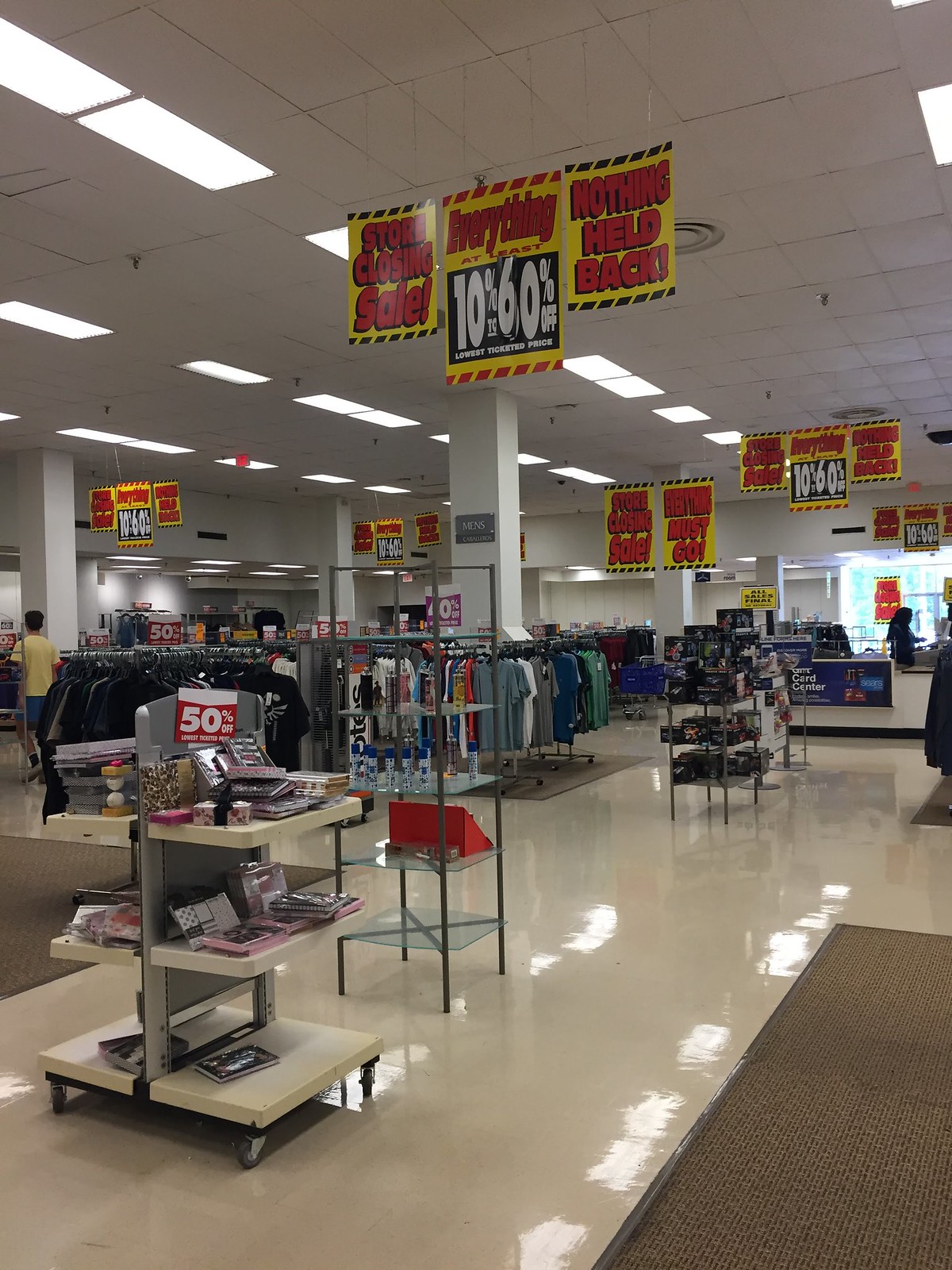The photograph captures the interior of a department store during a clearance sale. Prominent yellow and red signs proclaim "Everything Must Go," reflecting a sweeping liquidation. Suspended from the ceiling in the middle of the frame is a large sign indicating significant discounts, ranging from 10% to 60% off. The aisles, which once brimmed with products, now appear partially emptied as bargain hunters scour the remaining items. The floor, although not impeccably maintained, has been recently waxed, evident from its high sheen that effectively mirrors the overhead lighting.